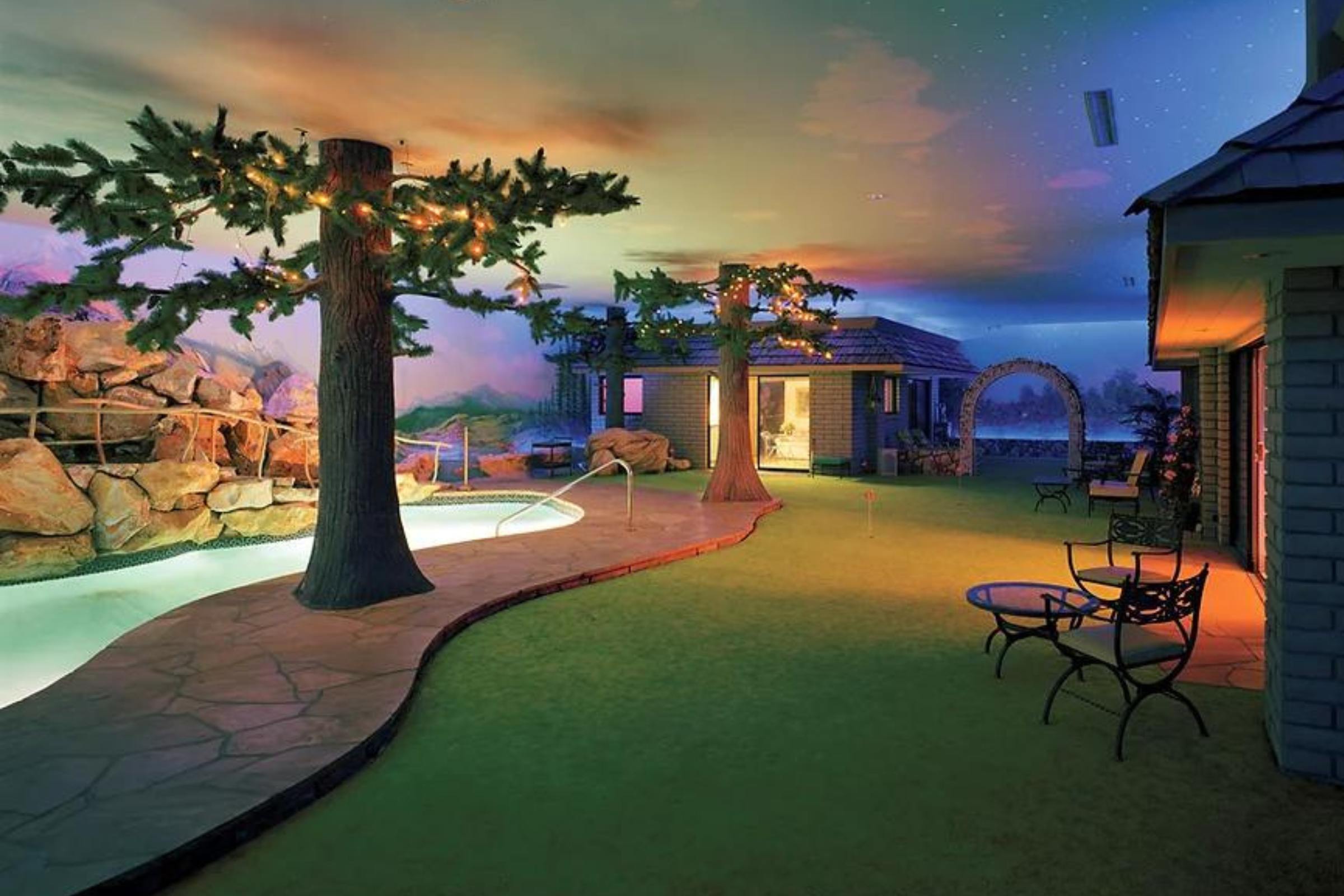The photograph depicts an indoor space meticulously designed and painted to resemble a picturesque outdoor setting. At approximately six inches wide and four inches high, the image offers a detailed glimpse into this creatively crafted scene. Starting from the left-hand side, a brown stone pathway meanders towards the center before curving back to the left, flanked by artificial trees with trunks extending up to the ceiling, adorned with branches and green leaves illuminated by small white lights. Adjacent to the pathway on the left is an in-ground swimming pool, bordered by a deck of faux stones and bricks, creating the illusion of a natural poolside area.

The ceiling is painted to mimic a sky transitioning from day to night as it moves from left to right, enhancing the outdoor illusion. On the right side of the image, the space features small mock houses with brick exteriors and sloped roofs, blending in seamlessly with the overall theme. One such house at the far right edge has a visible roof overhang, sliding glass doors, and emits light from within. Surrounding these structures are small round glass tables accompanied by chairs, placed on a green carpet that simulates grass.

In the background, an archway covered with ivy and a low stone wall add to the ambiance, while a cozy bedroom is visible inside one of the cottages. To the left of the pool, rock formations emulate a natural grotto, further extending the outdoor façade. Trees throughout the scene appear to be grounded in the artificial grass yet blend into the cloud-covered ceiling, giving the impression that the trunks disappear into the heavens. Overall, the photograph captures a whimsical and highly detailed indoor environment that convincingly transports viewers to an enchanted, outdoor-like fairyland.